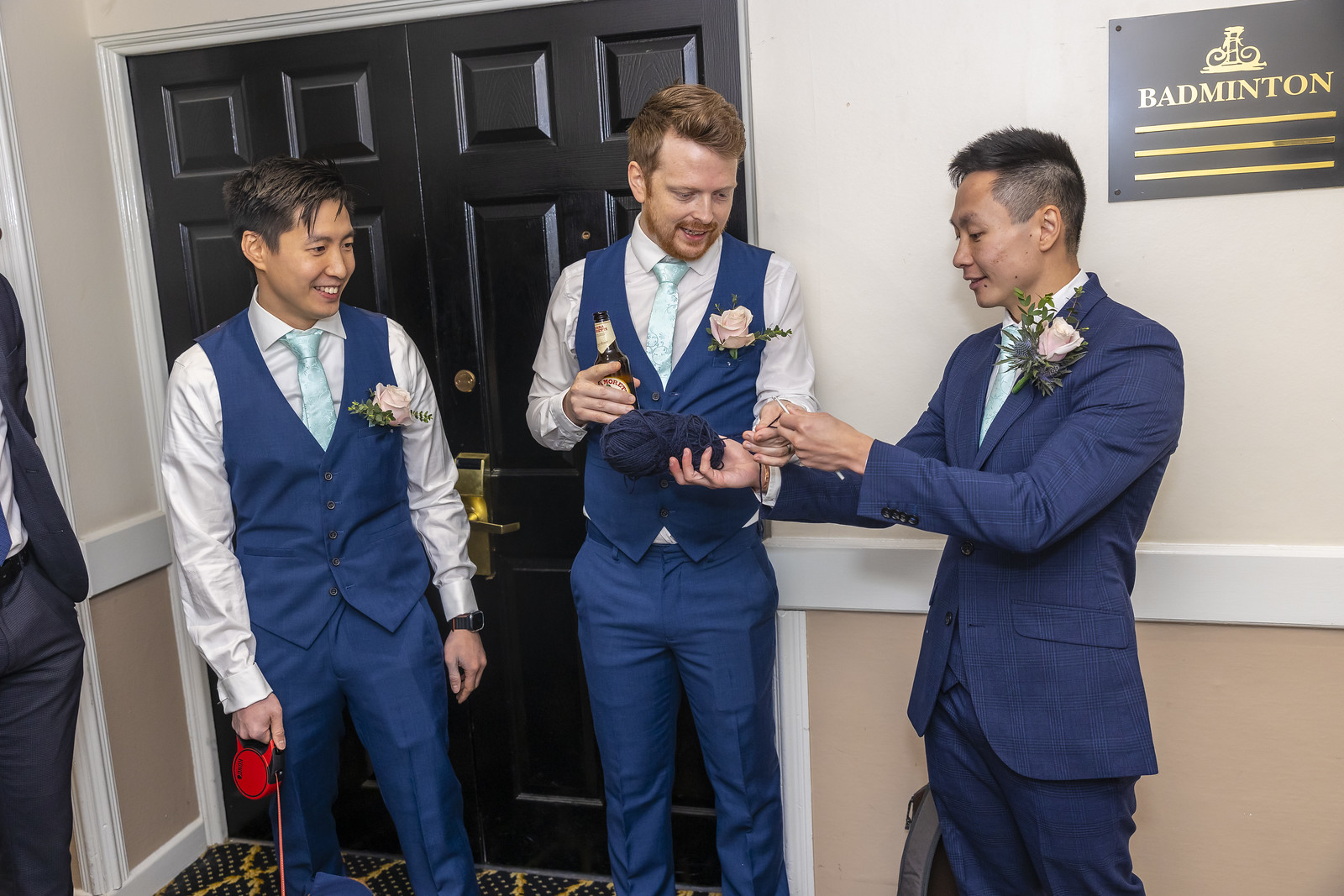In an indoor setting with light-colored upper walls and darker cream-colored lower walls, three men dressed in formal attire stand in front of double wooden doors, under a black sign with gold letters that read "Bad Benton" or possibly "badminton." The man on the right wears a royal blue jacket and pants, with a pink rose boutonniere pinned to his lapel and is holding a ball of yarn, showing it to the man in the middle. The middle man, with auburn hair and a beard, wears a matching blue vest and pants and holds a beer bottle in his right hand while intently looking at the threads of yarn in his other hand. The man on the left, smiling with black hair and wearing a blue vest, pants, and a white-collared shirt, appears to be holding a red dog leash, though no dog is visible. All three men are dressed similarly with light blue ties and rose boutonnieres, suggesting they could be part of a wedding party, possibly in a reception area.